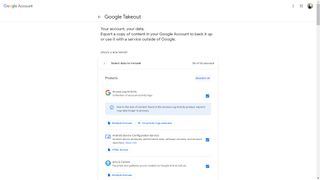In the upper left corner of the screenshot, the phrase "Google Account" is visible with the traditional Google logo in its iconic colors. On the upper right side of the page, there are three distinct icons, and an account icon is identifiable in the top right corner. The webpage appears blurry and the text is small, making it challenging to read.

A long scroll bar is situated on the right, featuring a light gray background and a medium gray section near the top, indicating the scrollable area. Towards the middle, faint text seems to read "Google Takeout," accompanied by an icon resembling a right-pointing arrow.

Below this, small black text is visible, with even smaller black text appearing like a headline on the bottom left of this section. A white rectangular strip with a light gray border is seen further down; the left side of this border appears slightly thicker than the right. Within this strip, bold or darker black text is noticeable, accompanied by lighter text on the far right.

Following another gray border, the word "Photos" is seen in black writing. Adjacent to this, there's a light blue rectangular background with darker blue text. At the very bottom, the Google "G" logo is displayed with two lines of black text to its right.